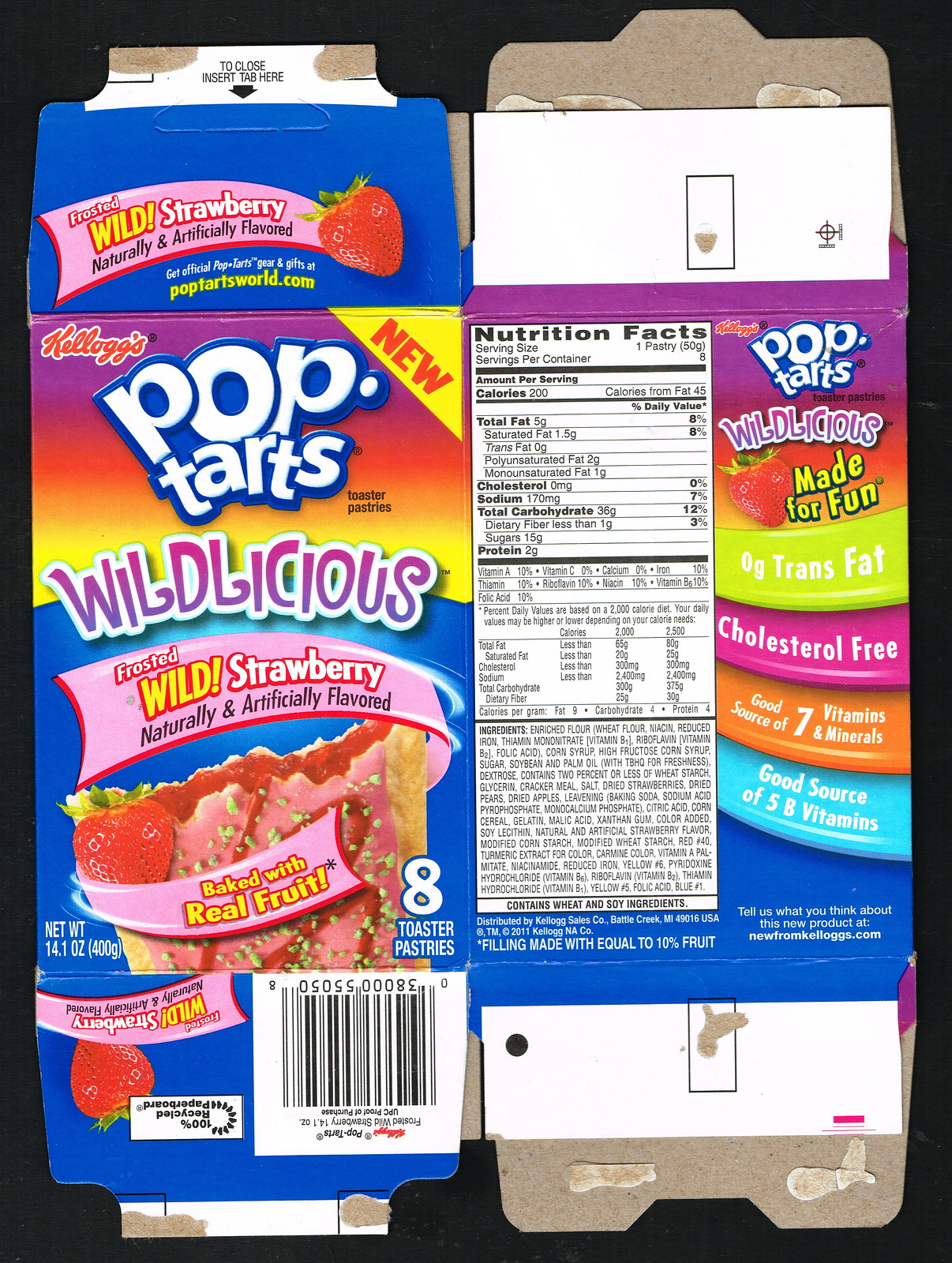This close-up photograph features a flattened, empty Pop-Tarts box against a black background. The box is vibrant and multicolored, showcasing a dynamic blend of purple, orange, yellow, and blue hues. On the left side of the image, the front of the box prominently displays the Pop-Tarts logo in bold white letters with a blue outline. Directly beneath the logo, the word "Wildlicious" appears in purple font. Below this, a striking pink banner proclaims "Frosted Wild! Strawberry," emphasizing the flavor with an exclamation point. An enticing visual of a half Strawberry Frosted Pop-Tart with colorful sprinkles adorns the area beneath the text.

On the right side of the image, another box panel reveals comprehensive nutritional facts printed in black on a white background. Additional nutritional highlights are listed against multicolored ribbons, stating: "Zero grams trans fat," "Cholesterol-free," "Good source of 7 vitamins and minerals," and "Good source of 5 B vitamins."